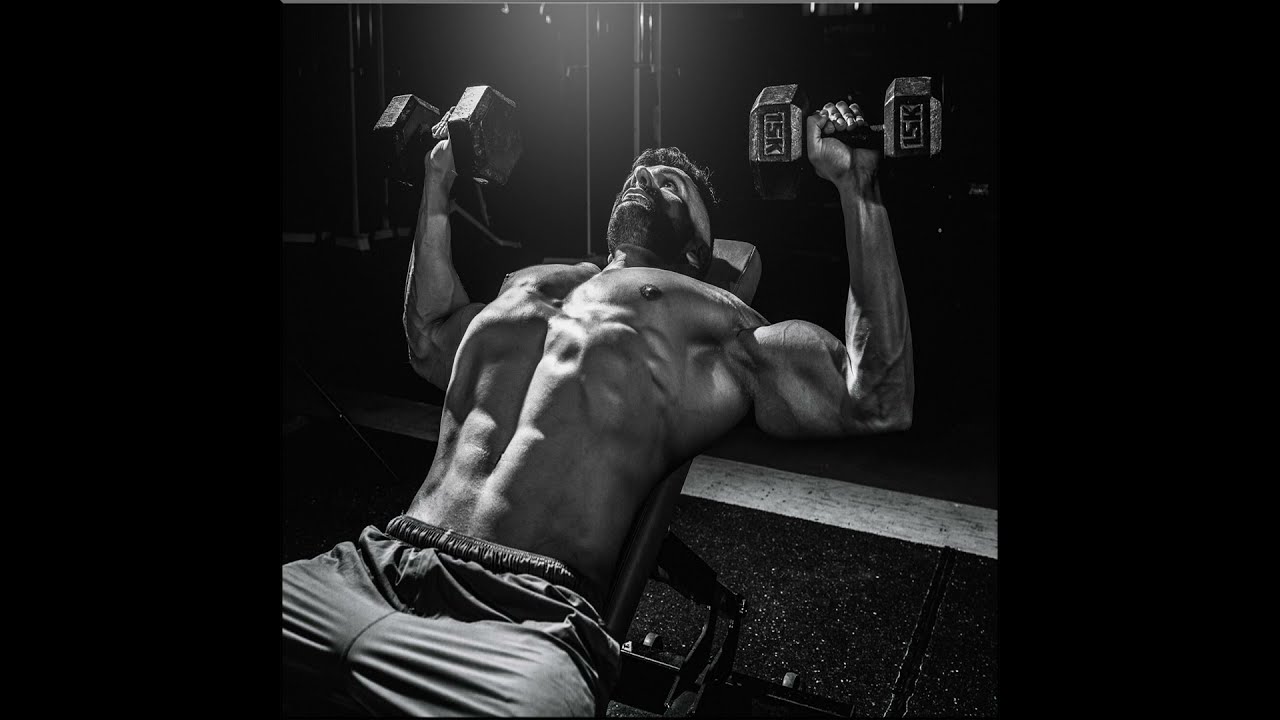This striking black and white photograph is framed by vertical black rectangles on each side, with the image itself centered in between. The photo captures a muscular man leaning back on a weight bench positioned at a 45-degree angle. He is seen from just above his thighs, which are visible in the lower left-hand corner of the image, upwards to his head. The man, who has brown hair and a light beard and mustache, is shirtless, revealing his defined upper body, including bulging arm muscles and a visible six-pack. He is wearing shorts with an elastic waist. Both his right and left hands are positioned out to his sides, bent at the elbows, each gripping a 15-pound dumbbell, lifting them in a chest press form. Above him, a light shines down, highlighting his muscular physique and the veins on his arms. The background features a mirrored wall, contributing to the intensity and focus of the scene. The floor beneath him is a black surface with a wood trim.